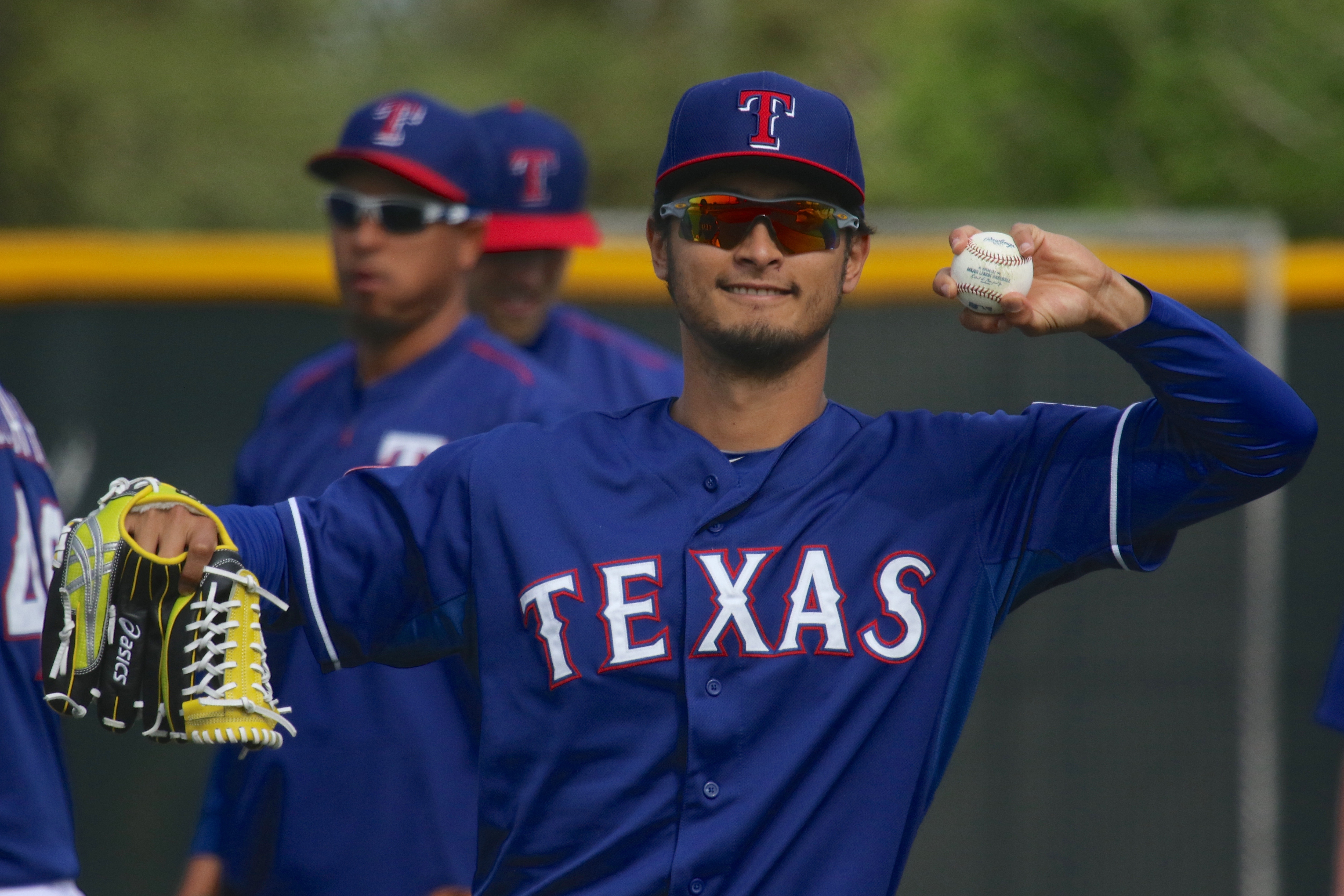The photograph showcases a professional baseball player from the Texas Rangers holding a bright yellow ASICS baseball mitt with black accents in his right hand and a baseball in his left hand. The player is dressed in a blue Texas Rangers uniform, which features "Texas" in white letters bordered by red. He is also sporting the team’s blue cap, marked by a prominent red "T" on the front. The background, slightly blurred, reveals other individuals and distant trees, suggesting the photo was captured in an outdoor, daytime setting under natural light. The image is sharp and detailed, except for the deliberately blurred background which enhances the focus on the player.